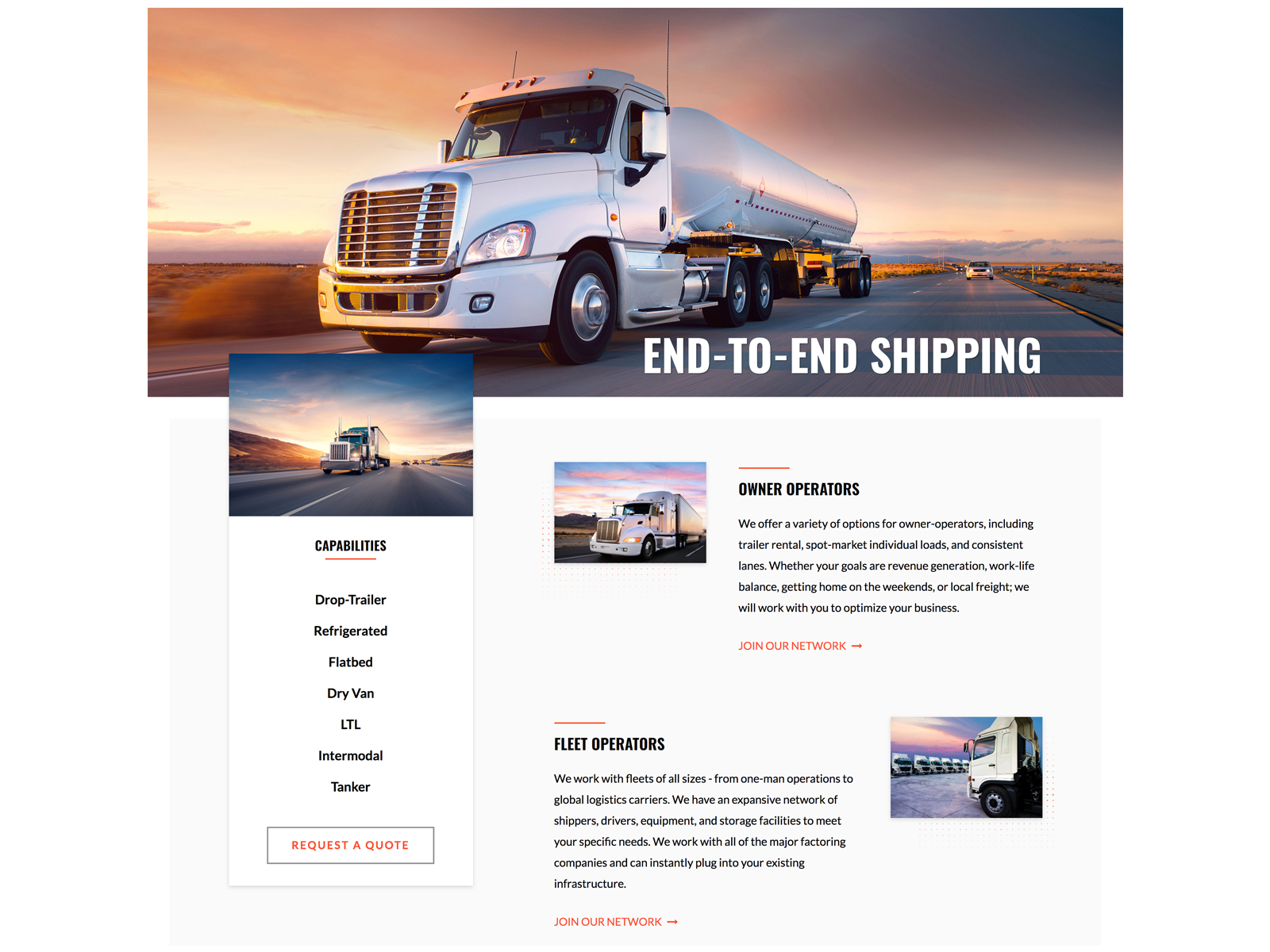A detailed image of a marketing advertisement for a trucking company, highlighting their comprehensive shipping and logistics services. The main photograph at the top depicts a large big rig truck with a cylindrical tank trailer, transporting liquids on a highway under a picturesque sunrise. The truck prominently features the text "End-to-End Shipping".

Adjacent to the main image, on the left, is a smaller yet similar photograph of another truck, also shown driving into the sunrise. Above this image, the caption "Capabilities" lists various shipping options provided by the company, including drop trailer, refrigerated, flatbed, dry van, LTL (Less Than Truckload), international, and tanker services. A "Request a Quote" button is visible below the list.

Beneath the main image, there is another photograph of a different big rig truck, accompanied by the header "Owner-Operators". This section details a variety of options available for owner-operators, such as trailer rental, spot market opportunities, individual load assignments, and consistent lanes. The text reassures potential partners that the company is committed to achieving various goals, whether they involve maximizing revenue, maintaining work-life balance, getting home on weekends, or focusing on local freight. The call to action encourages owner-operators to join the network.

Further down, the section labeled "Fleet Operators" explains the company’s flexibility in working with fleets of all sizes, from individual operators to global logistics carriers. Emphasizing an extensive network that includes shippers, drivers, equipment, and storage facilities, this part highlights the company's capability to meet specific needs and mentions their collaboration with major industry entities.